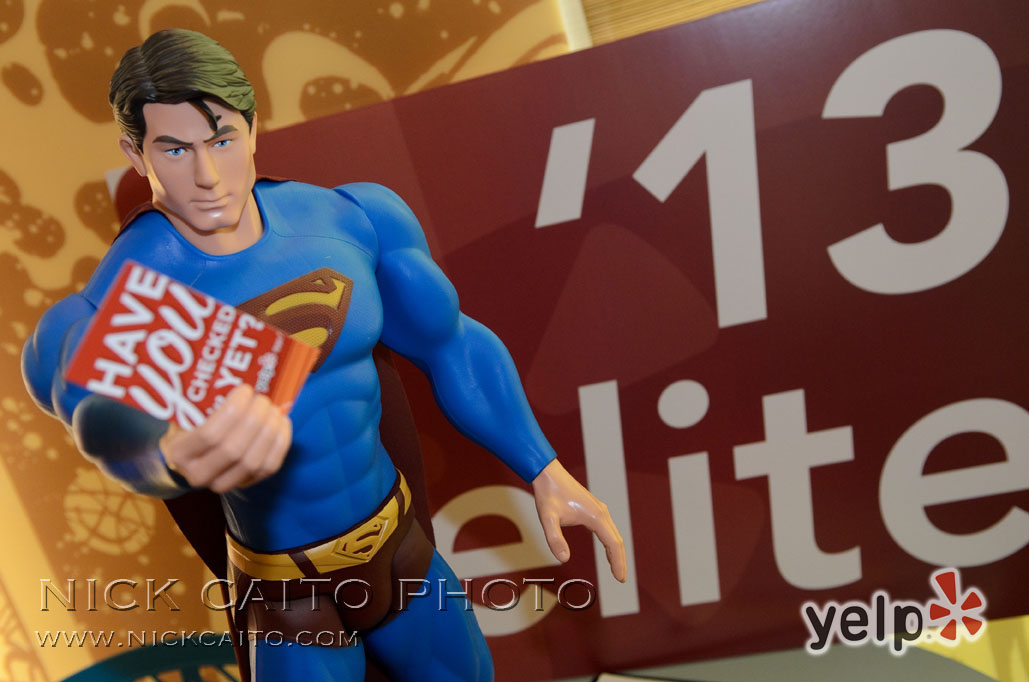The image is an indoor advertisement prominently featuring a Superman action figure. The figure is depicted in a typical Superman outfit, with a blue uniform adorned with the iconic "S" emblem on the chest, a gold belt, and blue pants over blue leggings. Superman is holding a red leaflet in his right hand that bears the white text, "Have you checked yet?" Behind the action figure, to the right, there is a card showing "13 elite" written in white on a red background. The bottom right corner of the image displays the Yelp logo, with the Yelp symbol in red, and on the left side, the photo is embossed with "Nick Cato photo" and the website "www.nickcato.com". Superman's hair is neatly swept back and gelled, adding to the classic look of the character.